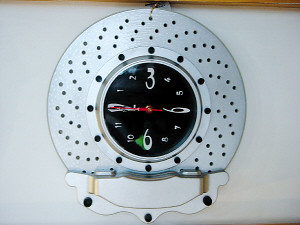This image features a circular clock displayed sideways within a square frame. The clock rests on a white platform, providing a stark contrast to its metal elements. Its outer rim, made of silver, includes evenly spaced holes around its border. The clock face is predominantly black, with white numerals arranged in a counterclockwise direction. Notably, the numbers 3, 6, and 9 are visible. The clock's single red hand stands out vividly against the dark background. Above the clock, a light brown object is partially visible but cropped out of the image frame.